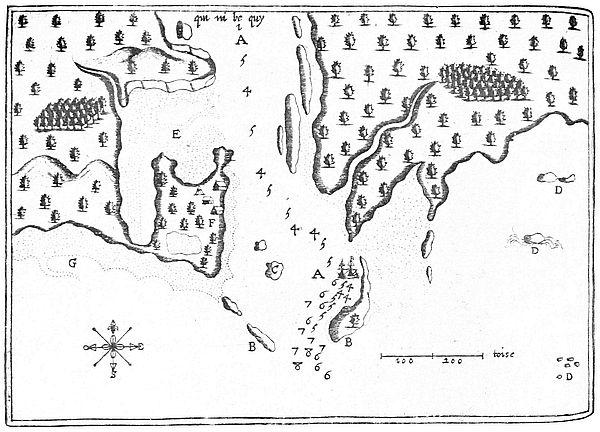This intricate black-and-white drawn map evokes an old-world style, possibly resembling a Gaelic map from the early 1500s or even a fantasy novel's depiction. Dominated by detailed pencil or grayscale illustrations, the map showcases various land areas and coastal features, including islands and bodies of water such as oceans and rivers that meander into them. Dense clusters of tree symbols scatter across the landscape, hinting at forests or orchards, while mountains add a touch of topographical variety. 

In the bottom left corner, a nautical compass orients the map with clear cardinal directions. The bottom right corner houses a distance measurement tool, designed to help gauge the scale of the map, though no specific legend is provided to decode the numbers 4, 5, 6, 7, and letters A through G scattered across the map. These annotations remain a mystery. The overall impression is one of a simple yet captivating map with a historical or fantastical allure, depicting a small, enigmatic coastal region.